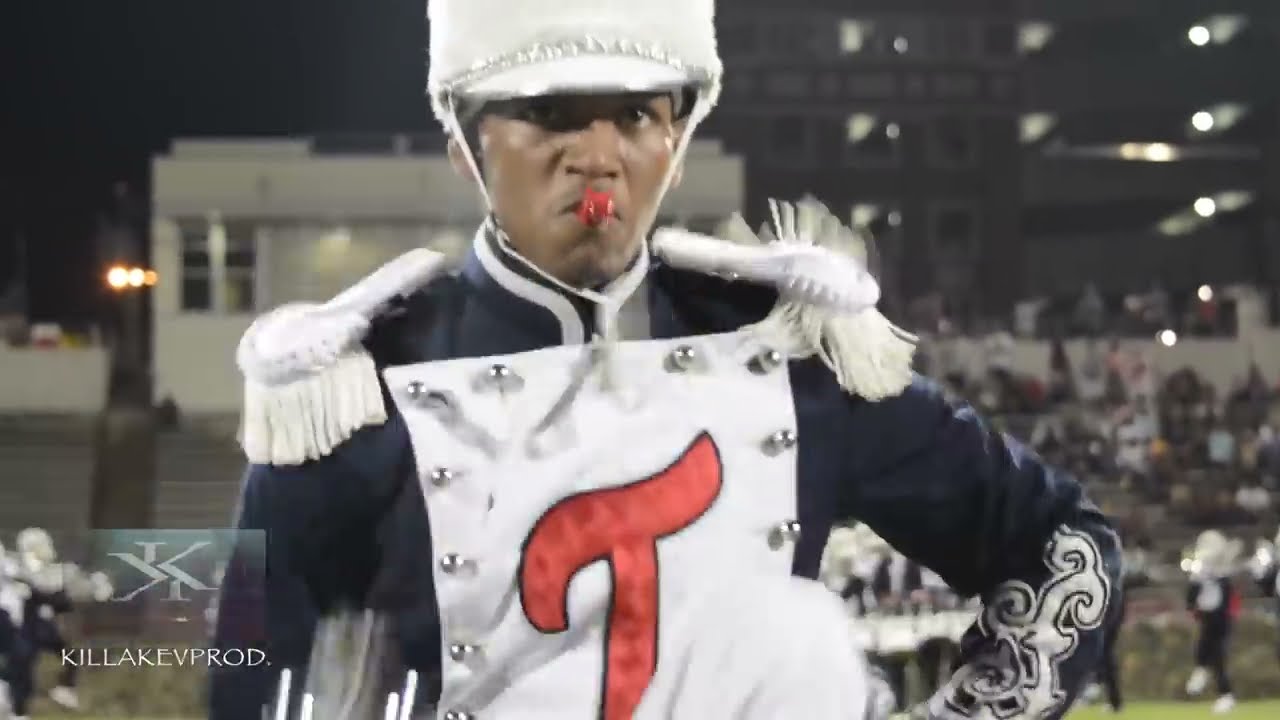The image features an outdoor scene of a diverse marching band performing on a green field. The band members are meticulously lined up in single file and are playing a variety of instruments, including tubas, trumpets, flutes, and trombones. They are all adorned in matching navy blue uniforms, which include pants and tops with white bib-like segments that have red lettering, though the specific text is obscured by their hands.

The band's headgear consists of large, cylindrical white hats featuring red and blue bands. The scene is set in front of a tan stone half-wall, behind which are stadium seating bleachers. The bleachers are occupied by a crowd dressed in a variety of colors including white, blue, yellow, orange, pink, gray, and black. 

The background shows the audience spread out and seated on silver benches with tan cement stairs running through the middle. The overall image appears slightly washed out, suggesting it was taken on an overcast day or is slightly overexposed. Notably, in the lower left corner, there is a watermark that reads "KILLEVPROD" with a stylized emblem featuring two K's, one forward and one backward.